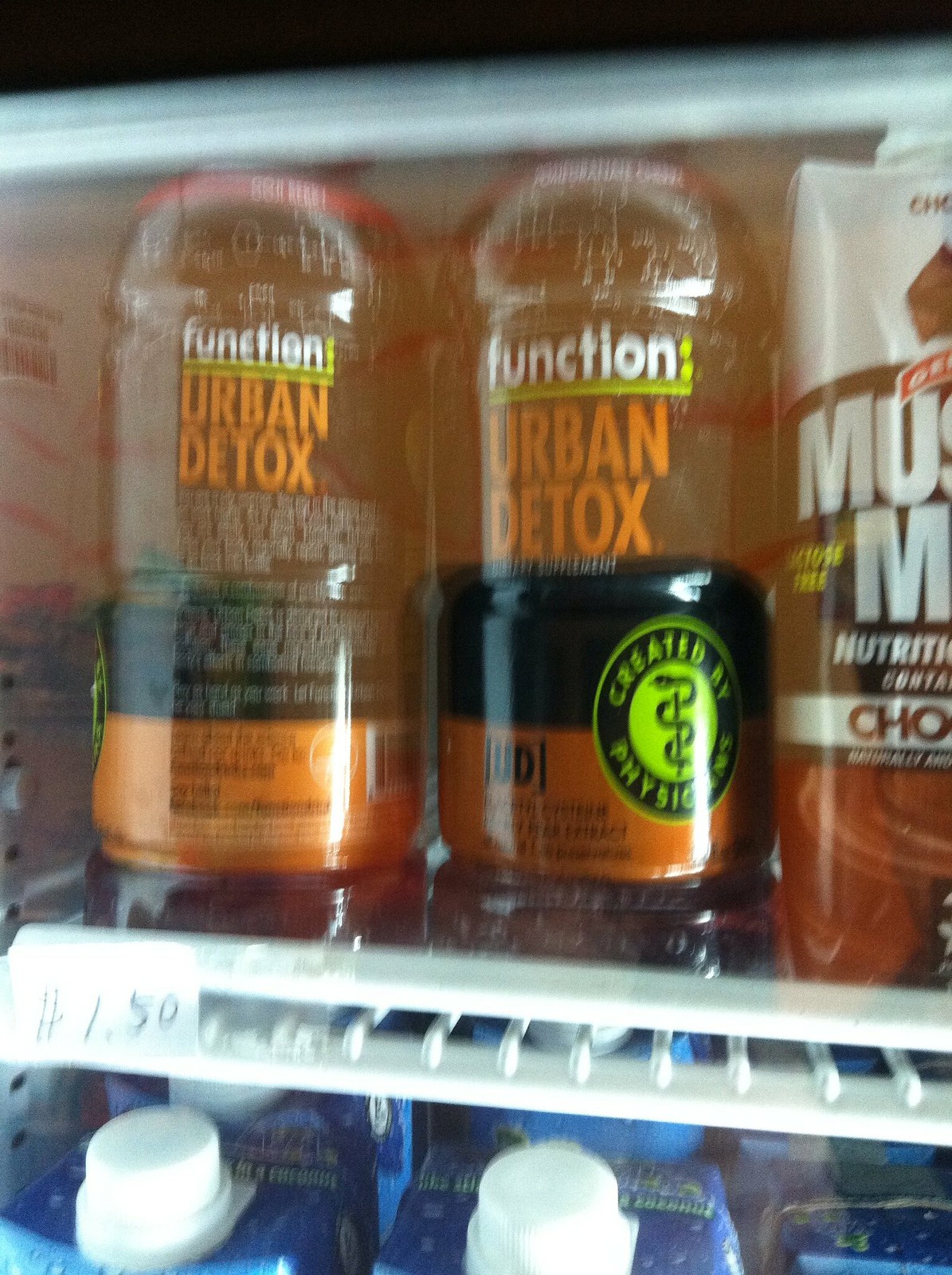An up-close photograph taken just outside the window of a vending machine, focusing intently on the first shelf. Dominating the frame are two bottles of "Function Urban Detox," notable for their packaging that prominently features the phrase "Created by Physician" in bold black and bright green text, along with a small snake emblem. Positioned adjacent to these bottles is a partially visible box of Muscle Milk. This packaging stands out with its white lid and with a combination of white and black segments, highlighted by chocolate-colored accents. The shelf below displays an array of blue-packaged items, each resembling a juice box. These items boast white lids and lettering, and the packaging is adorned with patterns that appear to be either snowflakes or water droplets. The arrangement shows three boxes prominently in the front, with a series of similar boxes extending into the background.